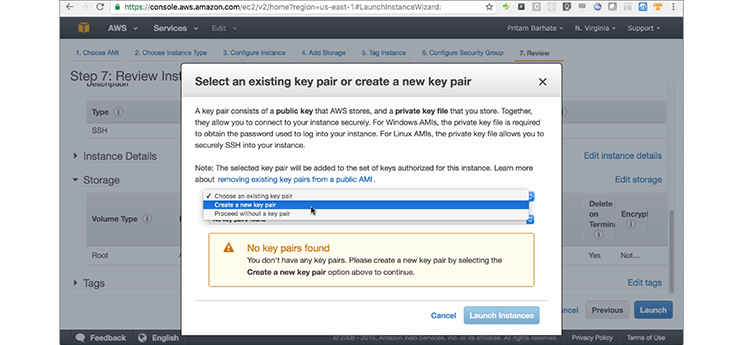The image is a detailed screenshot of the AWS Management Console displayed on a computer screen. At the very top, a white address bar indicates the URL "console.aws.amazon.com". Below the address bar is a black navigation area. On the left side of this black area, there is a yellow-colored box with the text "AWS" and a dropdown menu for services. Towards the right side, labels read "InVirginia" and "Support."

The main background screen displays a section titled "Step 7: Review Instructions." However, a white pop-up window prominently covers this section. At the top of the pop-up, a gray title bar reads, "Select an existing key pair or create a new key pair," with an option to close the pop-up (indicated by an 'X') on the right.

The main content of the pop-up is presented against a white background and explains the functionality of key pairs in AWS. It states:
"A key pair consists of a public key that AWS stores and a private key file that you store. Together, they allow you to connect to your instance securely. For Windows AMIs, the private key file is required to obtain the password used to log into your instance. For Linux AMIs, the private key file allows you to securely SSH into your instance. Note the selected key pair will be added to the set of keys authorized for the instance."

A clickable link offers additional information: "Learn more about removing existing key pairs from a public AMI."

Below this explanatory text, there is a dropdown menu where the user has opted to "Create a new key pair." An additional yellow-highlighted message in the pop-up informs the user that "No key pairs found. You don't have any key pairs. Please create a new key pair by selecting the Create a new key pair option above to continue."

At the bottom of the pop-up, a blue button labeled "Launch instructions" is visible, presumably guiding the user through the next steps.